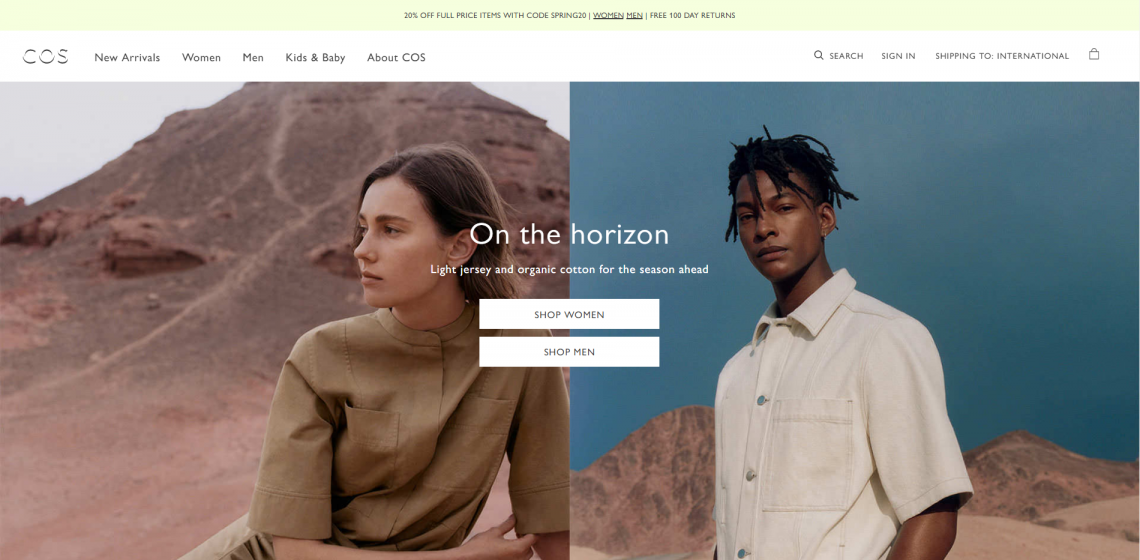This is a meticulously detailed computer screenshot featuring a stylishly designed website interface. Dominating the upper section is a white and pastel green rectangular header, centrally inscribed in black with minimal, finely printed text. To the left of this central text, displayed in white and outlined in gray, are the uppercase letters "C-O-S."

To the right of these letters, the navigation bar presents several options: "New Arrivals," "Kids & Baby," and "About C-O-S." Further right, a magnifying glass icon precedes the word "Search," indicating the search functionality. Adjacent to the search option, the interface lists "Sign In," followed by "Shipping to International" repeated twice for emphasis or possible design redundancy. Concluding this sequence is a shopping bag icon, suggesting the cart feature.

Below this header, the main body of the page is segmented into two adjacent images — one on the left and one on the right. Superimposed centrally on these images, both vertically and horizontally, are the words "On the Horizon" in white text. Beneath this, another white text line reads, "Light Jersey in Organic Cotton for the Season Ahead." Centered below this description are two prominent buttons labeled "Shop Women" and "Shop Men," inviting viewers to explore further. Each button corresponds with the picture it overlays: an image of a woman on the left and a man on the right, both styled to reflect the site’s aesthetic focus on organic cotton fashion.

This structured layout combines clean, minimalist design elements with clearly defined navigation options and a strong visual focus on sustainable fashion offerings.